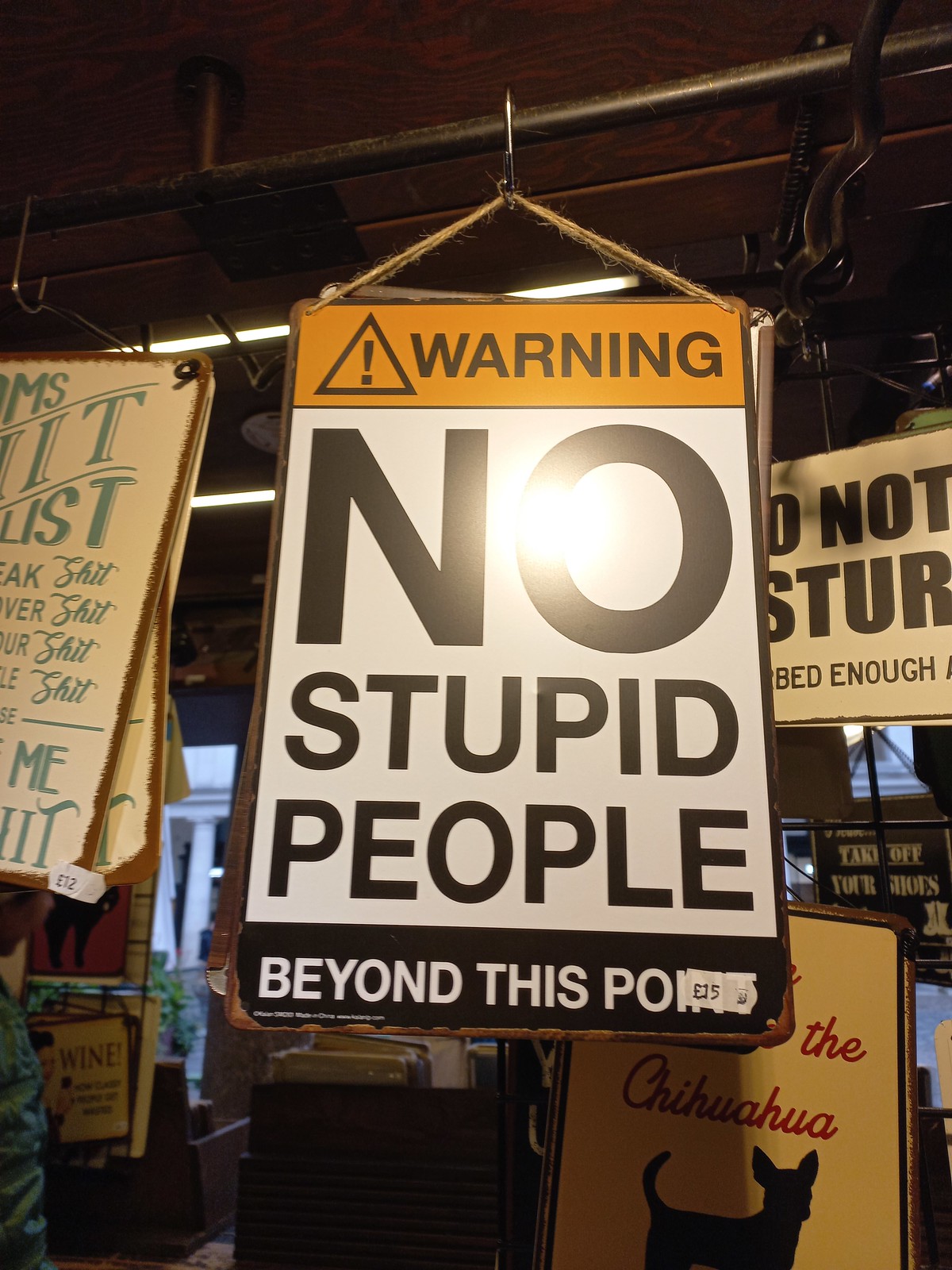In this color photograph, a prominently displayed sign captures the viewer's attention amidst an array of other partially visible signs in what appears to be a shop selling signage. The focal sign is suspended from a horizontal bar by a silver hook. At the top of the sign, a thick orange stripe features the word "WARNING" in capital black letters, accompanied by a triangular icon with an exclamation mark. Below this, against a white background, the phrase "NO STUPID PEOPLE" is boldly declared in large black capital letters. The bottom section of the sign has a black background with the words "BEYOND THIS POINT" in white capital letters. Additionally, on the bottom left of the sign, a label indicates the price as 15 pounds. Other signs are visible around it, but their messages are either obscured or partially cut off, featuring fragments like "chihuahua," "wine," and "do not disturb." The setting suggests a cluttered shop or warehouse ambiance.